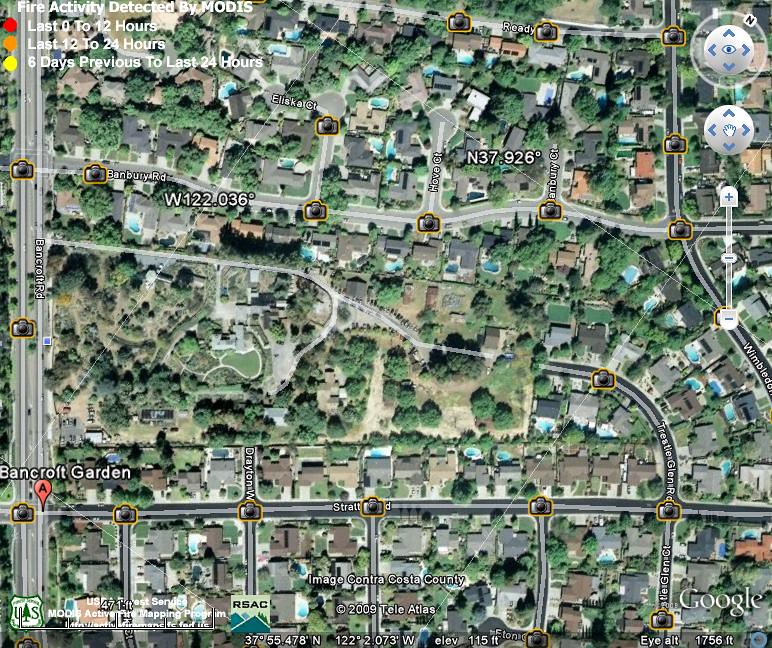An aerial view of a neighborhood captured using Google Earth's advanced settings, which allows users to see on-ground locations through embedded photographs. The image prominently features a fire activity alert from MODIS, indicating various levels of recent fire activity: red for the last 0-12 hours, orange for the last 12-24 hours, and yellow for 6 days previous to the last 24 hours. The coordinates displayed are west 122.036 degrees and north 37.926 degrees. A notable location on the bottom left is Bancroft Garden. The image encompasses several neighborhood areas and is annotated with "Contra Costa County" at the bottom, signaling it as a product of the United States Forestry Service map. Geographic coordinates are listed at the very bottom of the screen for detailed reference.